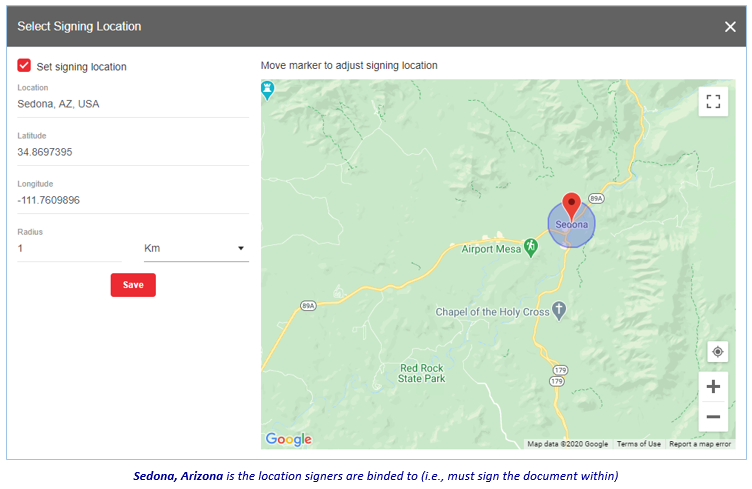This is a detailed description of an interactive map interface for searching and setting specific locations:

The top inch of the interface features a dark gray border with white lettering that reads "Select Signing Location" on the left side. On the right side of this border, approximately one-third of the way from the left, there is a white 'X'.

Below the top border, the interface is divided into two main sections. The left section contains a red box with a white checkmark and the text "Set Signing Location" in black. Below this box, there is a field to input the desired location, in this case, "Sedona, Arizona, USA." Beneath the location field, there are additional fields to enter the latitude, longitude, and radius. Centered on the left side, a red button with white text reads "Save."

The right section is predominantly occupied by a map. At the top of this section, a white strip displays the instruction "Move marker to adjust signing location." In the top right corner of this strip, there is a small blue location tab with a white piece in it.

The main map area shows land in teal, roads in yellow, and a prominent blue circle just right of center with a red location marker. Left of this circle, there is a small green tab labeled "Airport Mesa." 

In the top right corner of the map, there is a white square with black corner markings, and in the bottom left corner, there is a zoom control featuring a plus sign on top and a minus sign on the bottom to adjust the map's scale.

This comprehensive interface allows users to search for, adjust, and set specific geographic locations with precision.